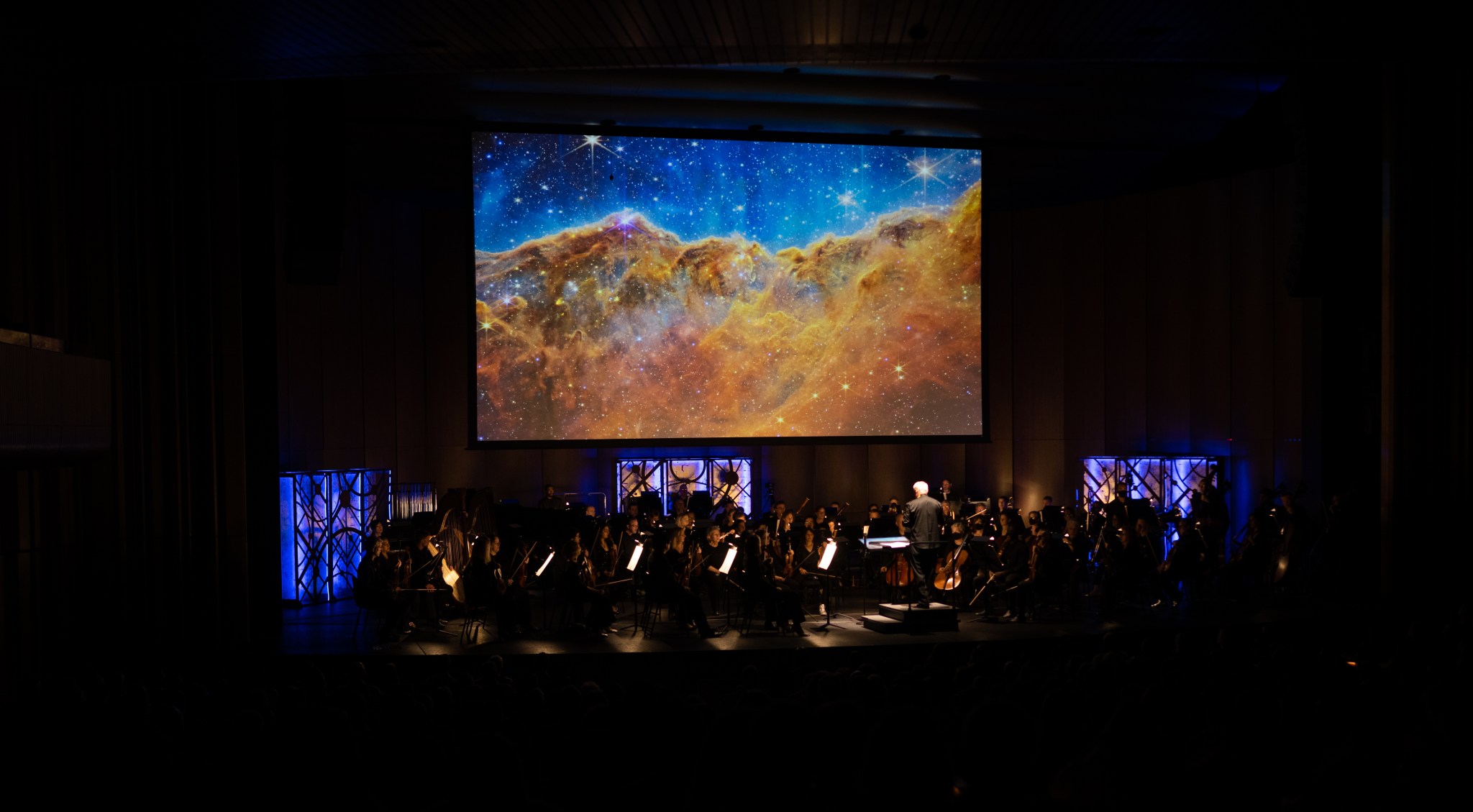The image depicts a dramatic, dimly lit theater stage where a full orchestra is performing. In the foreground, the conductor, distinguished by his white hair and illuminated podium, leads the ensemble of approximately 40 to 60 musicians, all dressed in black suits and attire, arrayed in several rows. The stage is enveloped in darkness save for subtle lighting that highlights key areas, creating a sense of mystery and depth. A massive screen dominates the background, displaying a striking space scene with stars, nebulae, and barren land reminiscent of images from the Hubble or James Webb telescopes. Purple and blue lights, strategically positioned at three points across the stage, cast an ethereal glow that enhances the space theme. This atmospheric image captured from the audience's perspective underscores a sense of immersive grandeur as the orchestra plays music synchronized with the celestial visuals on the screen.